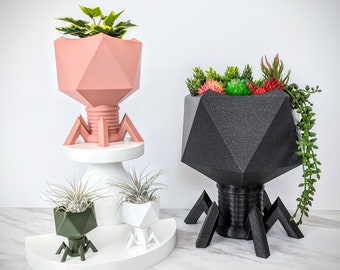The image showcases an advertisement for a set of abstract, insect-like plant holders of varying sizes, situated in a room with a white wall and a marble surface. The largest holder, colored black, is prominently positioned on the right and is adorned with vibrant succulents and green leaves. On the left, placed on a white riser, is a smaller light pink plant holder containing a lush green plant. Below this, a green and white mini holder displays air plants. Each holder features four legs and a unique topside design resembling a diamond or 3D cube. The background setting appears to be a cabinet or countertop, and the bright, colorful plants and elegantly crafted, six-legged plant holders create a visually striking and modern aesthetic.